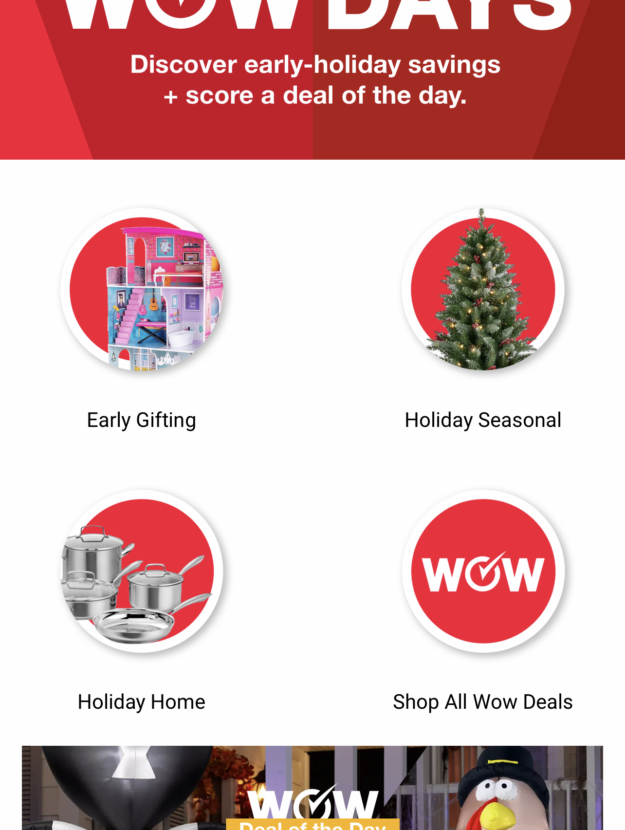Screenshot of a vibrant e-commerce website featuring a holiday promotion. The top portion is clipped, but partially visible is the "Wow Days" logo, characterized by a thinner "O" integrated with a checkmark, set against a red background. This logo appears intent on promoting early holiday savings and daily deals.

The midsection displays four prominent options arranged in a 2x2 grid, each within large, vividly colored circles with white borders:

1. The top-left circle is red with a white border and contains an intricate dollhouse image extending to the edge of the circle, accented by a subtle drop shadow. It is labeled "Early Gifting."

2. The top-right circle follows the same design layout but features a Christmas tree illustration and the label "Holiday Seasonal."

3. The bottom-left circle mirrors the others but showcases a set of three large silver pots and a pan, labeled "Holiday Home."

4. The bottom-right circle invites users to "Shop All Wow Deals," with the "Wow Days" logo centrally placed.

The footer, partially visible, teases a "Wow Deal of the Day" on a golden background, with only the upper portion of the text legible. Alongside this, a stuffed animal resembling a turkey and some autumn-themed decorations hint at a festive, fall atmosphere, indicating the promotion is likely for the early holiday and Thanksgiving season.